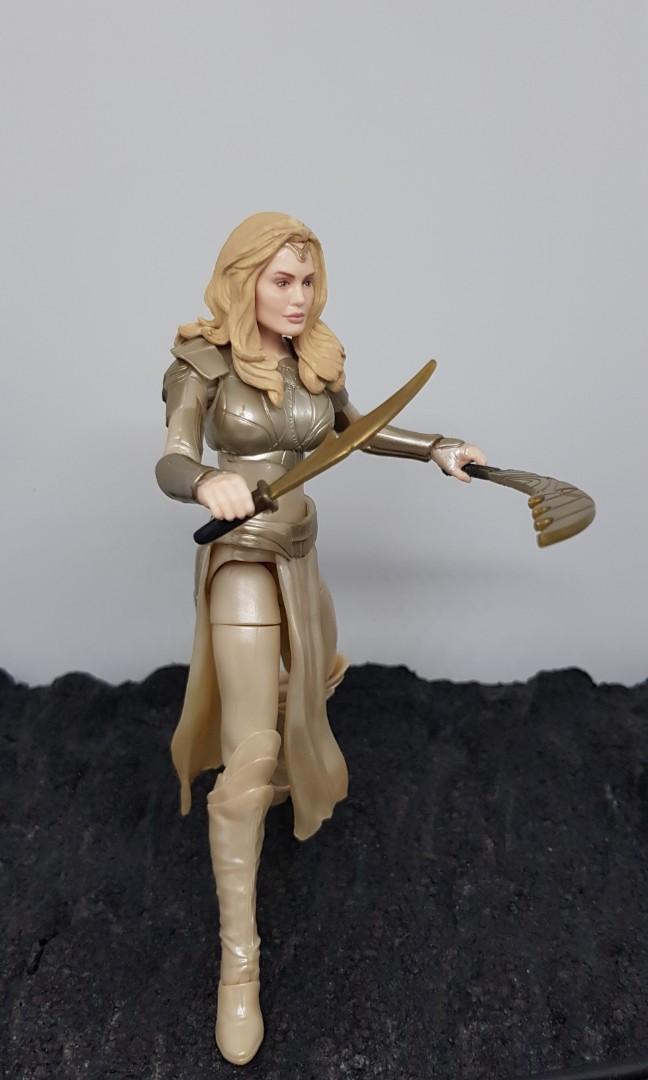This image features a detailed figurine of a white woman with long dark blonde hair, adorned with a triangular headpiece that rests on her forehead. She exudes a subtle, confident smile. Her attire is a combination of beige, bronze, and silvery armor, covering her upper and lower torso with a chest plate, shoulder plates, and gauntlets on her lower arms. The armor extends to a skirt-like garment from her hips to her knees, complemented by very light tan, knee-high boots. She is depicted wielding two weapons: in one hand, she holds a sword with a black handle and muted gold blade, while her other hand grasps a curved weapon featuring three gold elements on the blade. The figure stands on a black surface, with a light gray background that contrasts with her armor.